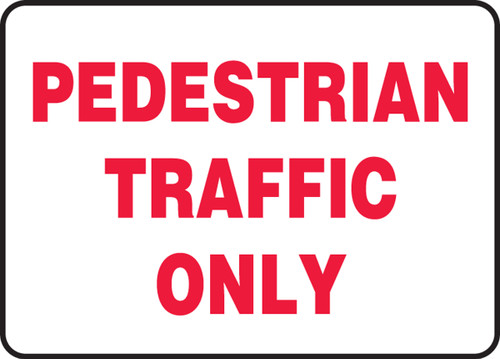The image depicts a rectangular sign with rounded edges outlined by a thin black border. The background inside the rectangle is white. Three words, written in capital letters and in red, are centered and stacked vertically from top to bottom: “PEDESTRIAN” at the top, “TRAFFIC” in the middle, and “ONLY” at the bottom. Each word is aligned centrally within the sign, and the entire design suggests that it is meant to indicate an area designated for pedestrian traffic only. The simplicity of the color scheme and layout emphasizes clarity and readability.